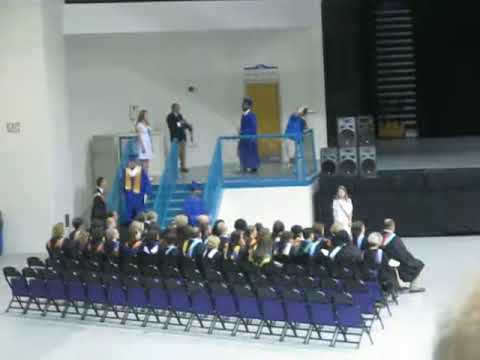This square photo captures a graduation ceremony taking place in an auditorium, featuring a stage with a gray floor and a black background curtain. The stage is set up with numerous stacked speakers on one side. A blue-railed staircase connects the stage to a landing, where people are walking up and down, including some graduates in blue gowns and caps. On the stage, a woman in a white dress and a man in a suit stand alongside one of the graduates. The setup includes about 50 to 75 metal chairs arranged in rows, with the front rows fully occupied by graduates. These graduates are wearing gowns, possibly black, with something draped around their necks, although the colors are not clear due to the image's blurriness. The rest of the scene includes white walls and a white-tiled floor, partially visible around the seating area.